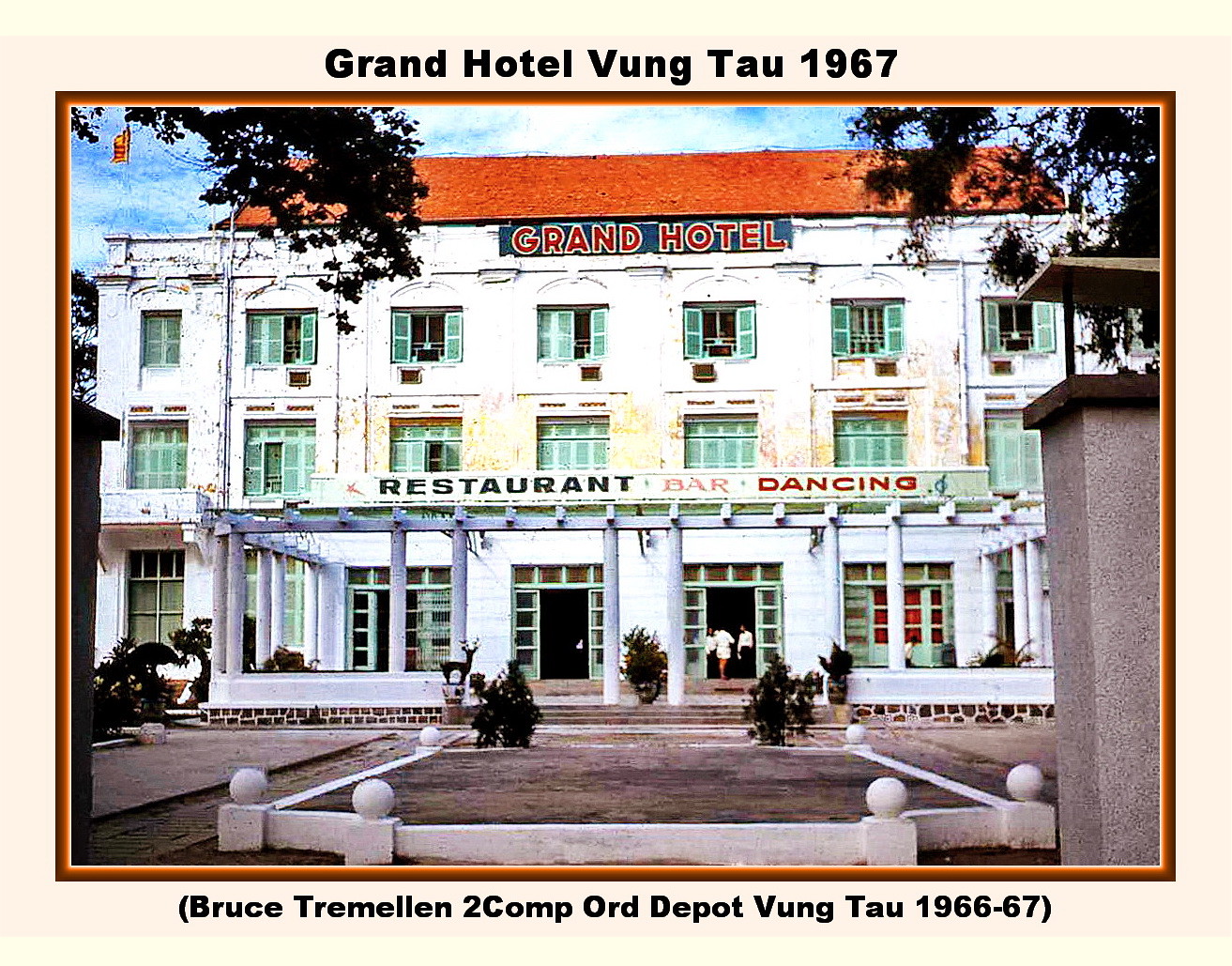This detailed photograph from 1967 shows the Grand Hotel in Vung Tau, Vietnam, surrounded by a light peach-colored border with black text. At the top, the text reads "Grand Hotel, Vung Tau, 1967," and at the bottom, in parentheses, it reads "Bruce Tremelin, 2 Comp Ord Depot, Vung Tau, 1966-67."

The Grand Hotel is a three-story, French colonial-style building with white walls and a red clay triangular roof. It features rows of windows with light mint green shutters on each floor. At the top of the hotel, a blue rectangular sign adorned with golden outlines displays the name "Grand Hotel" in bold, uppercase red sans-serif letters.

The ground floor showcases a grand entryway framed by numerous large white pillars. Above the entryway, a sign reads "Restaurant Bar Dancing" with "Restaurant" in dark green, "Bar" in pink, and "Dancing" in red fonts. The entrance consists of four doorways, each adorned with windows, leading into the hotel. Stone staircases ascend to the entry, enhancing its stately appearance.

In front of the hotel, there is a gray cement forecourt bordered by plant-filled areas. The scene is further accentuated by surrounding trees with dark green leaves. This image captures not only the architectural details but also the historical essence of the Grand Hotel during the mid-1960s.